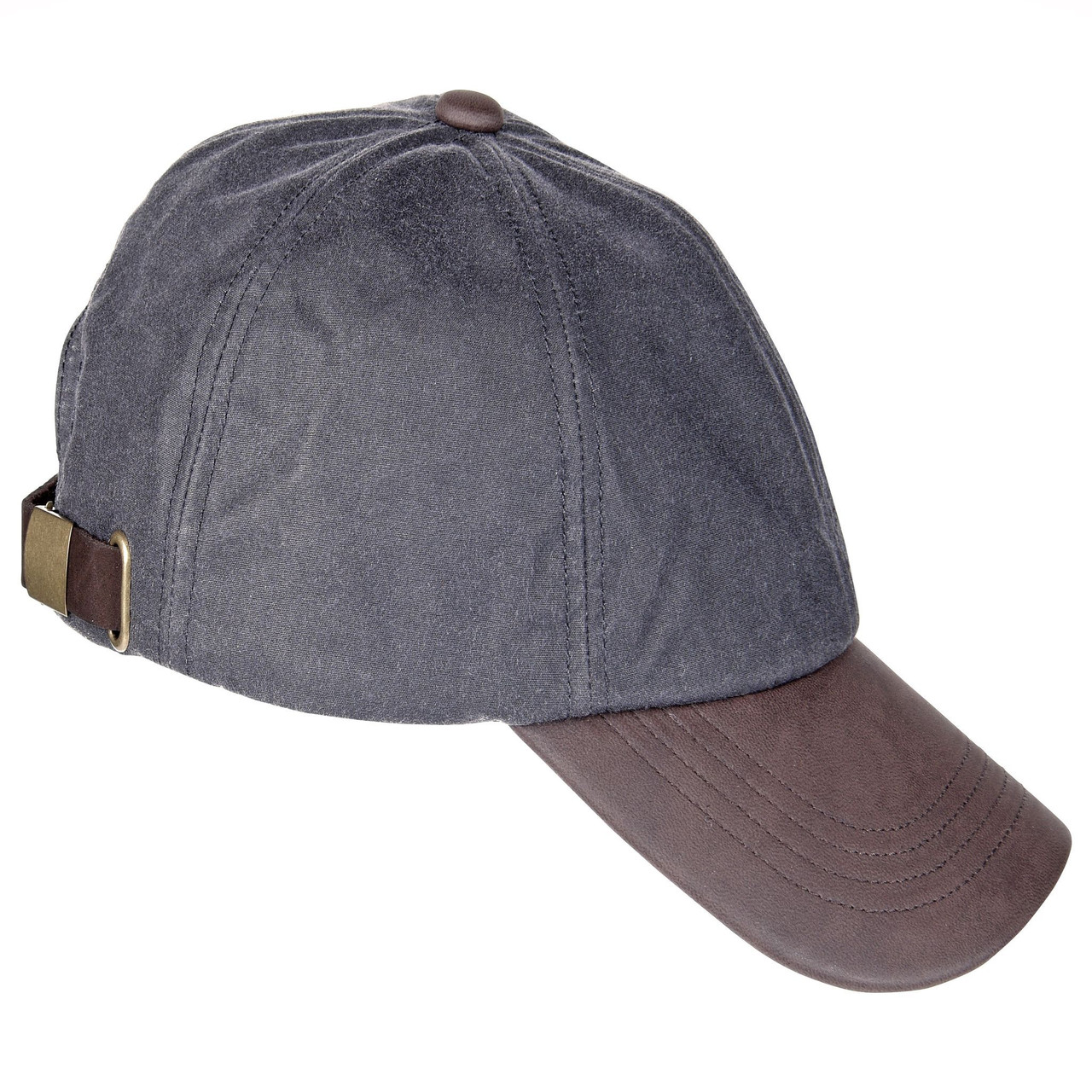This image is a detailed, up-close view of a baseball-style cap, isolated against a pure white background, likely edited to emphasize the hat. The cap appears in a real photograph, probably shot on a green screen with the background removed. The main part of the hat is a faded grayish color with visible seams and a brownish button at the top that has a slight mauve hue. The bill or peak of the cap, which features four-stitch lines, is similarly brown with mauve undertones and exhibits a leather-like appearance. At the back, there's a brown leather strap for size adjustment, secured with a gold-colored clasp, adding a touch of sophistication. The overall quality of the cap suggests it could be well-suited for a product photo, perhaps intended for use on an e-commerce website, despite lacking any brand iconography. The hat is shown at a side angle, highlighting its detailed craftsmanship and material textures.